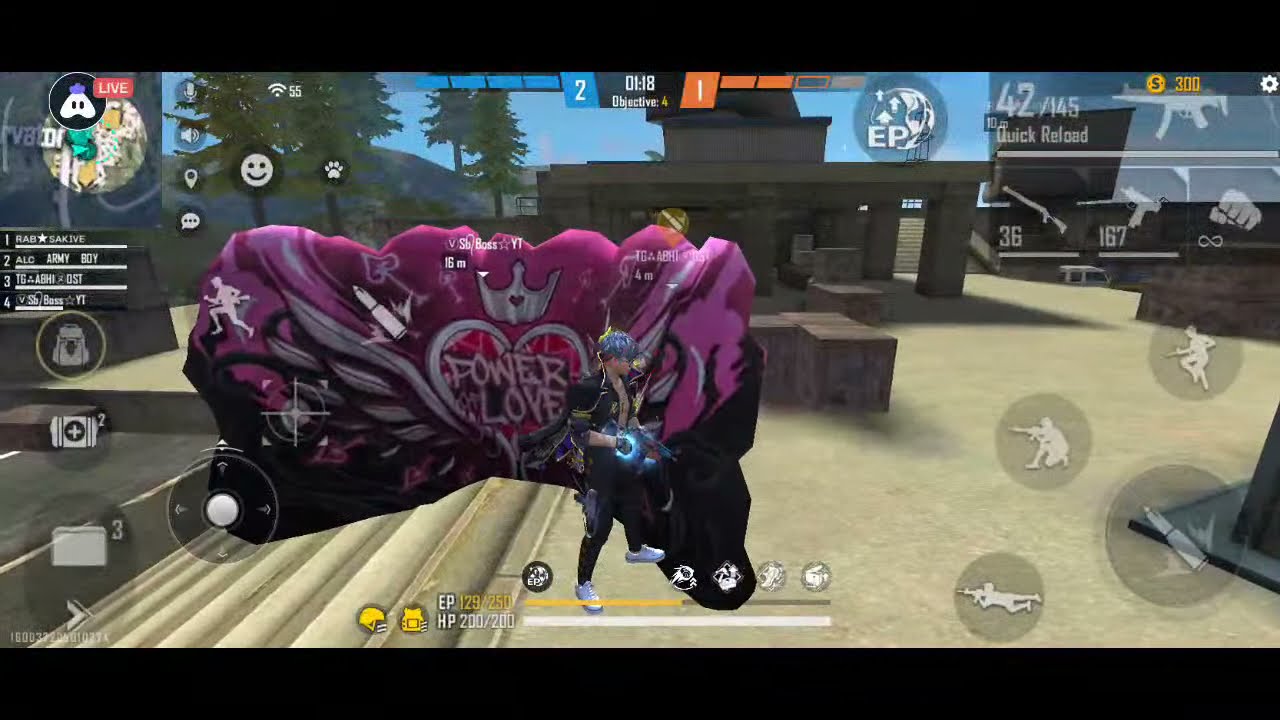The image is a screenshot from a video game, possibly a PC game, featuring an outdoor scene with a character prominently displayed in the foreground. The character, a man with blue hair, is dressed in a black outfit with an open jacket revealing no shirt underneath, dark pants, and white sneakers. He is holding something glowing blue, which appears to be a weapon. Behind him stands a graffiti-covered rock wall with vibrant purple, pink, and black colors, showcasing the words "Power Love" alongside a red heart and a crown. In the background on the left side, there are trees under a blue sky, and to the right, there is a building. The top left of the screen displays the word "Live" with a status icon and a list numbered 1 to 4, possibly indicating players in the game. The top right corner shows "142/145" and "quick reload," likely representing ammunition count alongside a weapon icon. Additionally, icons of people in different positions holding guns are visible in the lower right corner, suggesting various player statuses or actions. Framing the top and bottom of the image are black rectangles, indicating a dynamic and action-packed gaming interface.